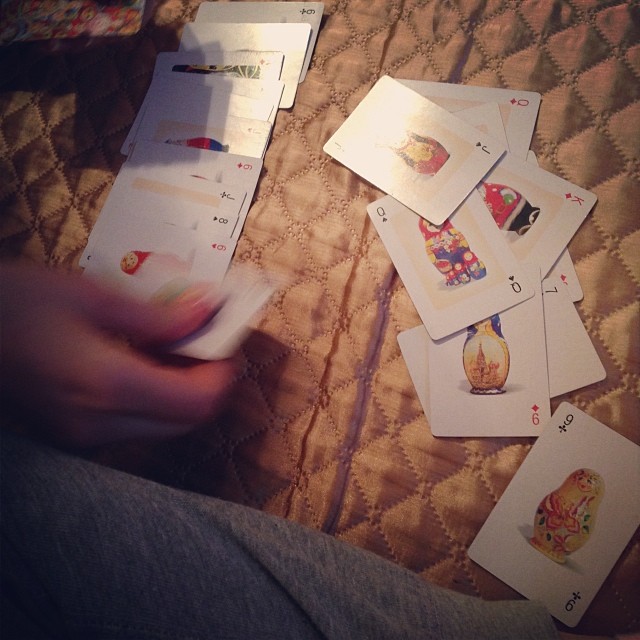In the image, a group of people is engaged in a lively card game atop a bed. The bed features brown, shiny checkered bed sheets or a blanket, giving a distinctive backdrop to the scene. A hand, clad in gray sweatpants, is seen in motion, moving a card. The scattered cards on the bed display an array of figures: the jack, queen, king, nine, six, and eight. Each card showcases a unique toy-like figurine. For instance, the nine displays a yellow figurine with a facial expression and intricate body decorations, while the queen card features a figure adorned with a red headdress, yellow hair, and distinct attire. The detailed designs on each card contribute to the vibrant and playful atmosphere of the card game.